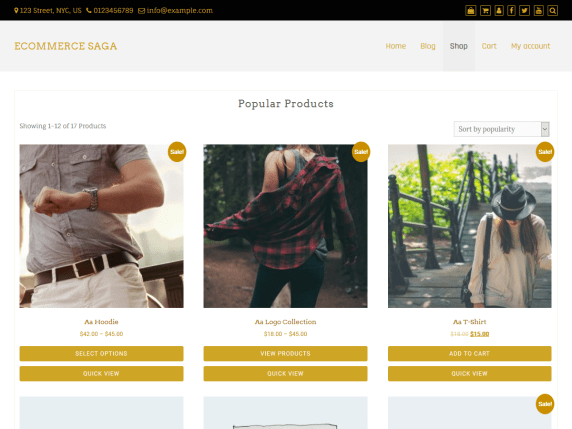The image showcases a desktop computer screen displaying a website titled "E-Commerce Saga." At the very top, a thin, hardly readable black bar spans across the screen. Below this is a prominent gray header featuring the site’s name in bold, followed by navigation tabs labeled "Home," "Blog," "Shop," and additional, indistinct options. The "Shop" tab is active and distinguished by its black color, while the others are highlighted in gold.

Beneath the header, a section titled "Popular Products" is visible, presenting three main product images. The displayed content indicates "showing 1 of 32 products," though only three pictures are shown. The first image depicts a man checking his watch, with his head out of frame, leaving visible only his pants, belt, and shirt. The second image features a woman with her back turned, dressed in black jeans or leggings, a flannel shirt, and an off-the-shoulder top. The third image shows another woman walking upstairs, donning a long sweater, a hat, and carrying a purse while looking downward. 

Directly below these images are gold buttons linked to various products available for purchase, suggesting that the current category focuses on clothing items.